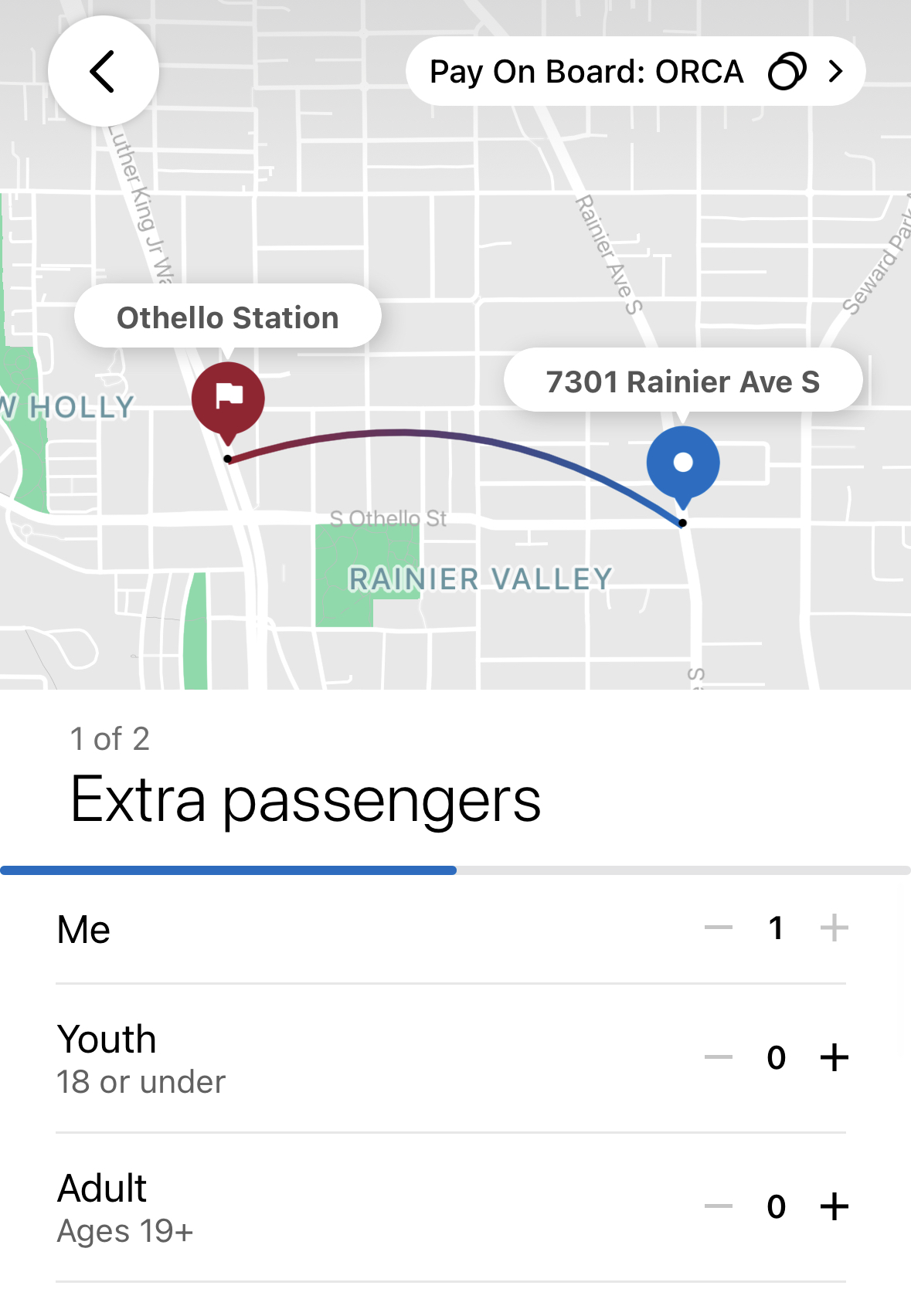**Detailed Caption:**

This is a screen capture from a rideshare app interface displayed on a smartphone. At the top of the screen, there is a status bar featuring a left-facing back arrow on the left side, indicating a back button, and on the right side, there is a "Pay-On-Board ORCA" option accompanied by a right arrow. Below the status bar, the main section of the screen shows a map highlighting various locations. Prominently marked on the map is a red bubble with a white flag labeled "Othello Station." 

Additionally, a blue circle on the map indicates the user's current location, identified as "7301 Rainier Avenue South." Various streets and neighborhoods are visible on the map, including Rainier Valley, South Othello Street, and Martin Luther King Jr. Way. 

Beneath the map section, an interface allows the user to adjust passenger details. A blue-grey progress bar labeled "Me" is partially filled, suggesting a seating or service status. Below this bar, options for adding extra passengers are provided. These include fields for "Youth 18 or under" and "Adult ages 19+," featuring the option to input number values using plus and minus buttons, all initially set to zero.